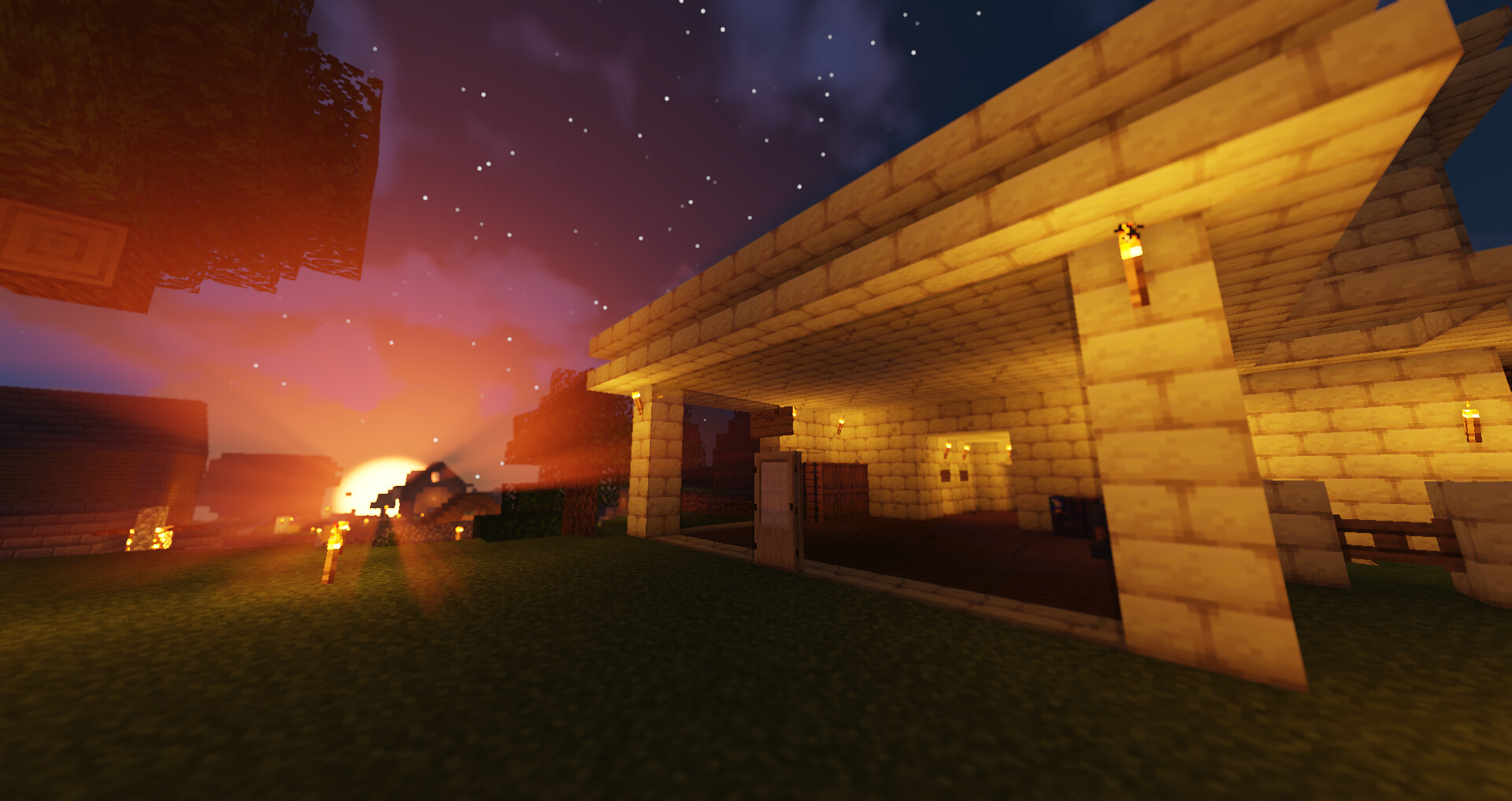This image is a detailed still from the video game Minecraft, enhanced with mods or possibly AI to create a surreal atmosphere. Dominating the middle of the scene is a sandstone structure, composed of tan "block bricks," which features several torches emitting light and mounted both on the walls and the surrounding grassy area. The building has an entranceway that appears to be open or perhaps with a glass pane that's not immediately visible, revealing the interior.

On the left side, there's a traditional Minecraft tree crafted from square blocks with green foliage and a single "branch" distinguished by darker edges and two shades of tan in the center. Various other structures, constructed primarily from tan wood with dark brown roofs, populate the background, contributing to the bustling settlement atmosphere.

The sky, a vivid gradient ranging from deep blue to pinkish-purple-red, is marked by numerous white dots resembling stars, enhancing the nighttime scene. Unlike the usual blocky design of Minecraft, the sky displays realistic-looking clouds and a large, circular yellow sun either setting or rising on the horizon. This sun's presence, coupled with the night sky, adds an otherworldly touch as the traditional Minecraft sun is square.